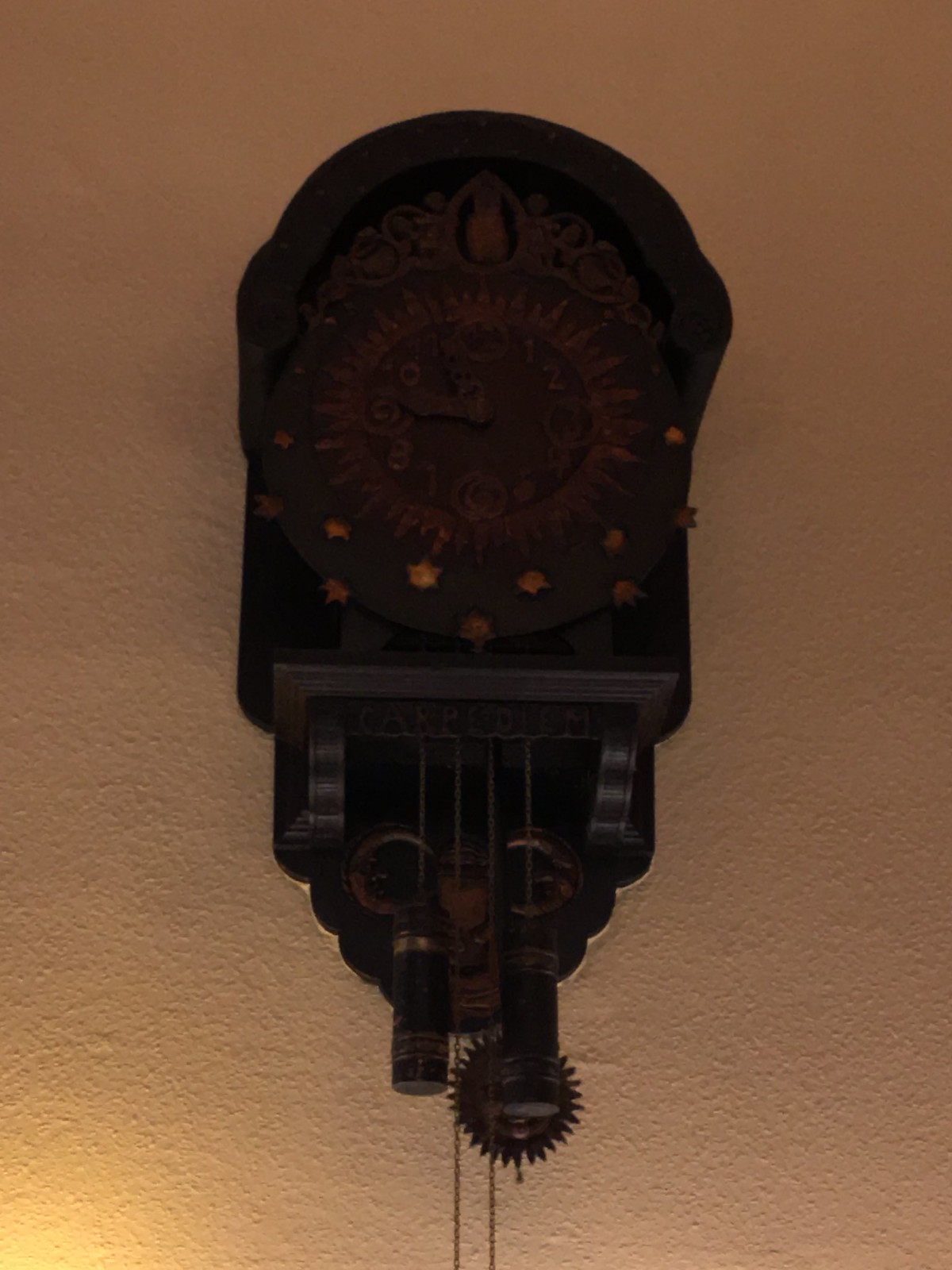The image depicts an antique clock, shrouded in darkness due to the lack of flash during the photography. The clock appears to be mounted either on a wall or hanging from the ceiling. Despite the poor lighting, one can faintly discern the outlines of the clock's face, including small lines where the numbers would typically be, as well as its hands. The clock features an unconventional design; while the upper part resembles a traditional clock, the lower portion exposes its intricate mechanical components. Visible gears and other mechanisms dangle from the bottom, showcasing the inner workings of the timepiece. A subtle shadow of these components is cast on the wall. In the bottom left-hand corner of the image, a tiny speck of light suggests the presence of a lamp, possibly placed on a nearby table, gently illuminating the scene.